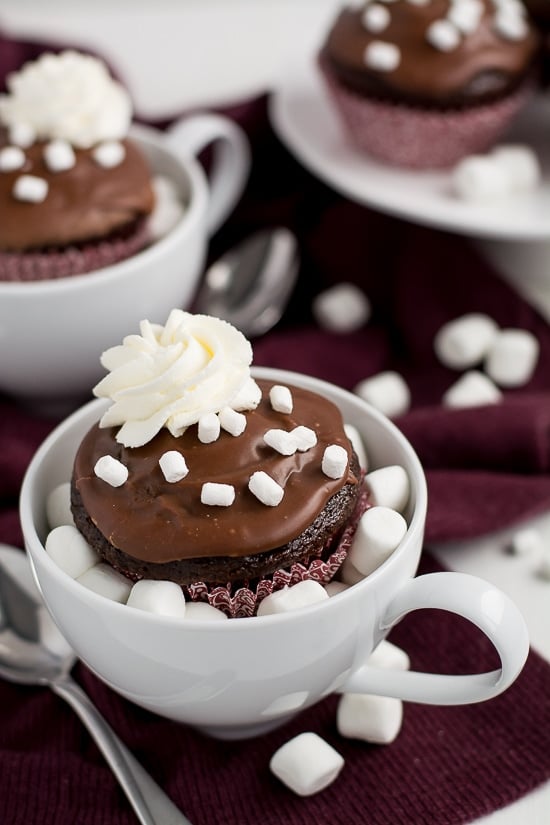The image showcases a tantalizing arrangement of chocolate cupcakes and marshmallows artfully presented in white mugs. Central to the composition is a white mug holding a chocolate cupcake adorned with rich chocolate frosting, a delicate white frosting rosette, and an array of small white marshmallows both on top and surrounding the cupcake within the mug. To the left of this is a silver spoon, adding a touch of refined elegance. The scene extends into the background where an identical white mug houses another similarly decorated chocolate cupcake amidst marshmallows. Completing the visual feast, a lone chocolate cupcake with tiny marshmallows perched atop sits on a white plate in the upper right corner. These delectable treats are set on a maroon tablecloth, noticeably bunched and dotted with scattered white marshmallows, providing a warm contrast that highlights the array of whites, browns, and silvers within the image. The handle of the primary mug is positioned to the right, anchoring the composition centrally, while the arrangement of the other items adds depth and a sense of indulgent abundance.